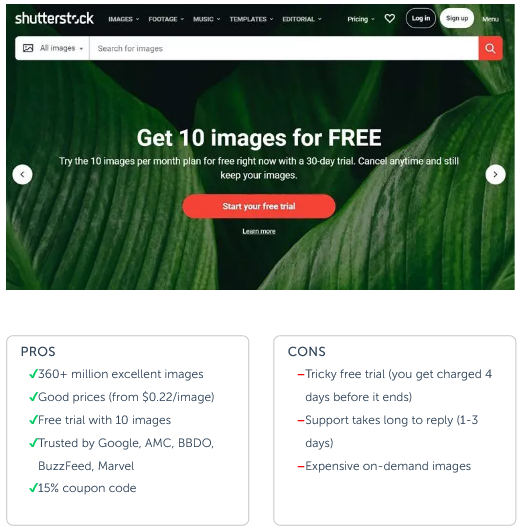The home page of Shutterstock prominently features a close-up image of green leaf tips, highlighting the detailed ridges of approximately five leaves. At the top of the page, a navigation bar in white text spans from left to right and includes the company name "Shutterstock" followed by various categories: "Images," "Footage," "Music," "Templates," "Editorial," and "Pricing," each accompanied by a drop-down menu. Additionally, there is a heart icon for favorites, a white-outlined oval labeled "Log In," and a solid white oval labeled "Sign Up," with the word "Menu" located in the upper right corner. Below the navigation bar is a long white rectangular search bar with a dropdown option for "All Images" and a search field for images.

Centered beneath the search bar is a promotional message: "Get 10 images for free. Try the 10 images per month plan for free right now with a 30-day trial. Cancel anytime and still keep your images." Adjacent to this message is a prominent orange oval button labeled "Start Your Free Trial" in white text, followed by a smaller "Learn More" link in white text.

Further down, a comparison table outlines the pros and cons of the service. On the left, the pros include "360+ million excellent images," "good prices starting from $0.22 per image," "free trial with 10 images," and the endorsement "trusted by Google, AMC, BBDO, BuzzFeed, Marvel," as well as a note about a "15% coupon code." On the right, the cons listed are a "tricky free trial" that charges you four days before it ends, "support takes long to reply (1-3 days)," and "expensive on-demand images."